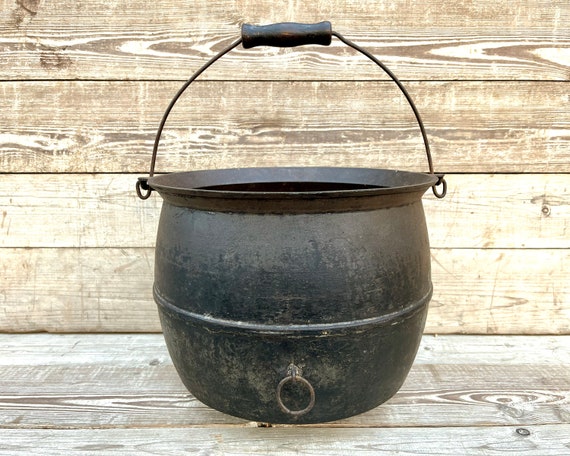This photograph captures a well-weathered, barrel-shaped black cast iron pot, resembling an old cauldron. The pot's surface is significantly textured and aged, with patches where the black has worn down to reveal a brownish patina, indicating long-term use. A thin wire handle arches from side to side above the pot, with a thicker black metal grip at the center, making it easier to carry. Additionally, a small metal ring is attached to the front lower section of the pot. The pot is placed on a light wooden surface, likely made of planks, which matches the wooden panels in the background. The panels on the back wall align horizontally, creating a cohesive rustic setting that gives the entire scene a simple, yet timeless, charm.